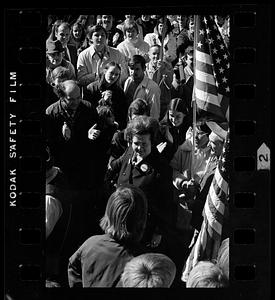The image appears to be a vintage black and white photograph, likely from the 1960s or 70s, captured as a section of a negative on Kodak Safety Film, with the text "Kodak Safety Film" running vertically up the left side and a number '2' contained in an arrow on the right side. It shows a group of approximately 20 people standing outside on what seems to be a sunny day. Central to the image is a woman who resembles Margaret Thatcher, the former Prime Minister of the United Kingdom. She seems to be the focus of attention, possibly signifying a political gathering or event. Two American flags are prominently displayed on poles behind her, suggesting the setting is somewhere in the United States. The people in the image are clad in attire and hairstyles typical of the era, adding to the photograph's historical context.